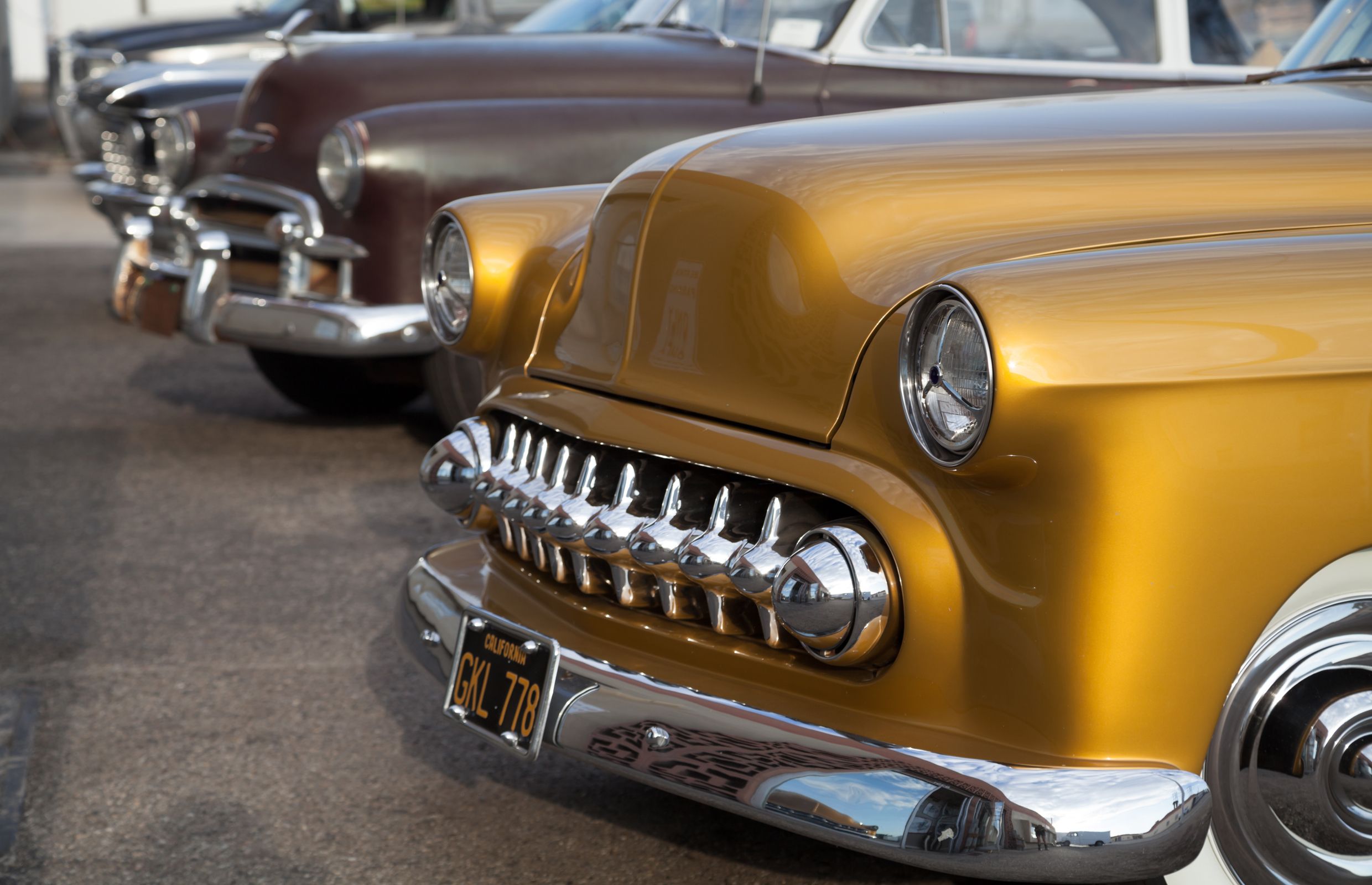The photograph depicts a vibrant lineup of classic cars parked outdoors on a concrete surface, likely at a car show under daylight conditions. The most prominent vehicle in the foreground is a meticulously polished gold 1930s-era car, featuring a gleaming chrome grille and bumper. The license plate reads "California GKL778" in yellow font set against a black background. Directly behind it is a car in a brownish-red color, bearing similar chrome accents and appearing almost identical to the first. Further back, although increasingly blurry, there are additional vehicles, one of which is a dark gray or black car. The clarity of the image diminishes with each successive car, emphasizing the detailed craftsmanship of the foremost golden vehicle.